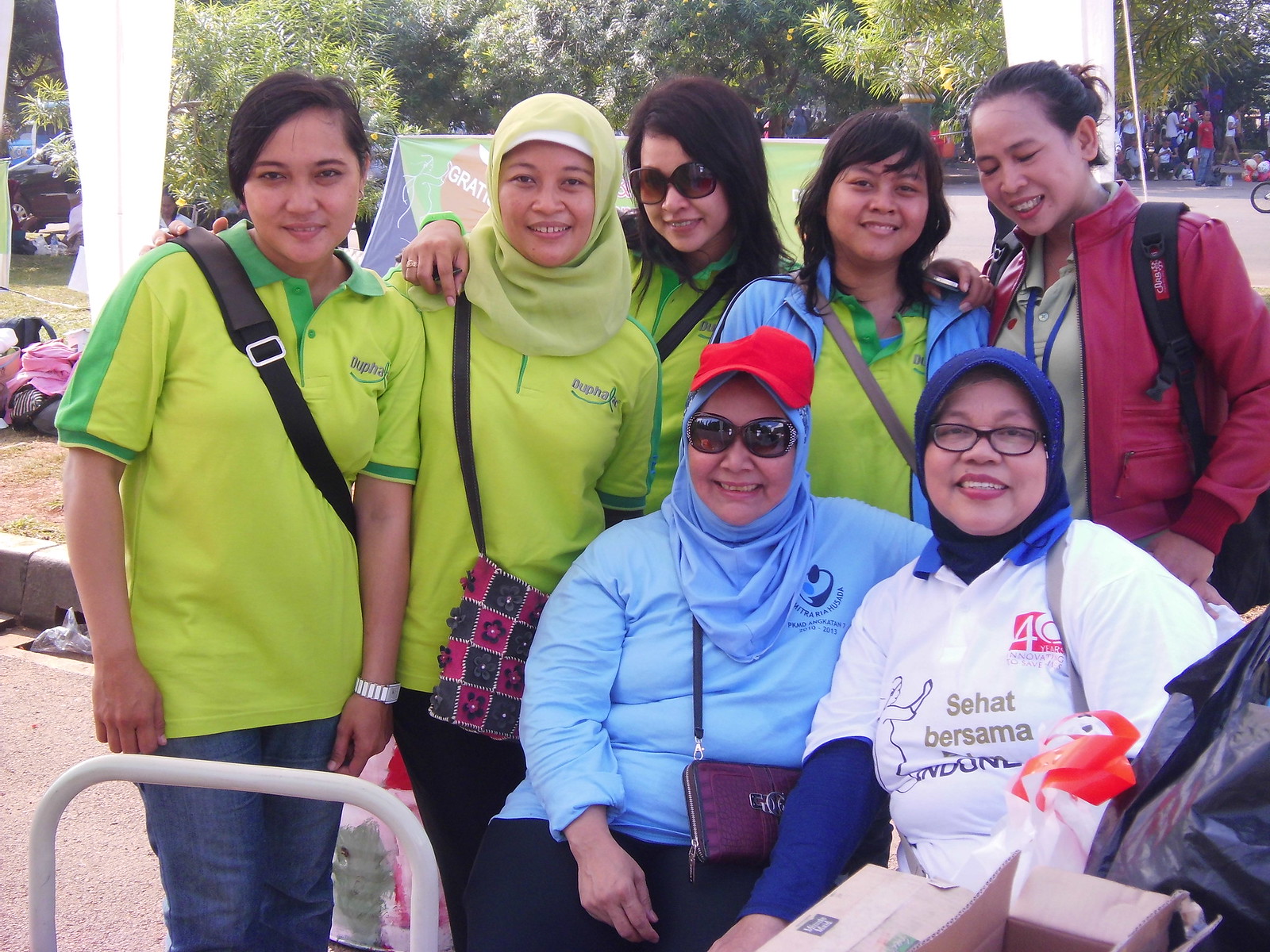In this image, set in a sunny outdoor location that appears to be a public park with a sandy surface, seven Asian women, possibly Filipino, are posing directly in the center of the frame. The setting is enriched by the presence of numerous trees in the background and bustling activity with several people faintly visible further back. The women are dressed in diverse outfits: four of them don lime green shirts resembling football jerseys, and three are wearing hijabs, indicating they might be Muslim. Among the rest, one woman is in a white shirt, another in a blue shirt, and another in a green shirt with a red jacket. Details such as one of the women having "Seahawks, Burisma" and the number 40 on her shirt are discernible. All the women have purses slung over their shoulders, and three of them are wearing glasses, with two pairs being shaded against the bright midday sun. The scene is vivid with a palette of colors including white, brown, tan, various shades of green, black, silver, pink, red, and blue. The image is devoid of any text beyond the mentioned apparel details and includes a few objects like a pole and what seems to be an open box or some equipment in the foreground. The women are smiling and posing, creating a warm and cheerful atmosphere.